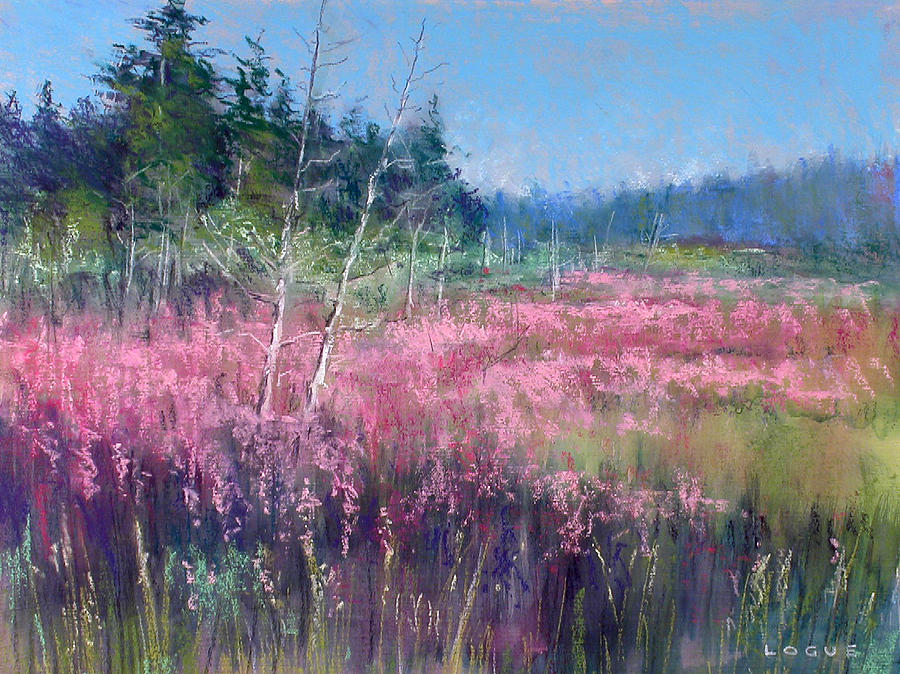This oil painting by the artist Logue, whose signature is clearly displayed in white capital letters at the bottom right corner, depicts a serene and untouched outdoor landscape. The scene features an expansive field filled with tall, green grasses and clusters of pink, red, and purple flowers, with hints of yellow and green interspersed throughout. In the foreground, white birch-esque trees stand prominently among the vibrant flora. The middle ground showcases a thicket of evergreen trees rising above the field's edge, while in the distance, a mix of taller trees and possibly mountains create a soft, fading backdrop. The sky above is a delicate blue with wispy gray clouds, contributing to the painting's soft, pastel color palette and overall glowing, dreamlike quality. The use of the dry brush method results in the soft lines and somewhat blurry details, emphasizing the painting's ethereal and peaceful atmosphere.